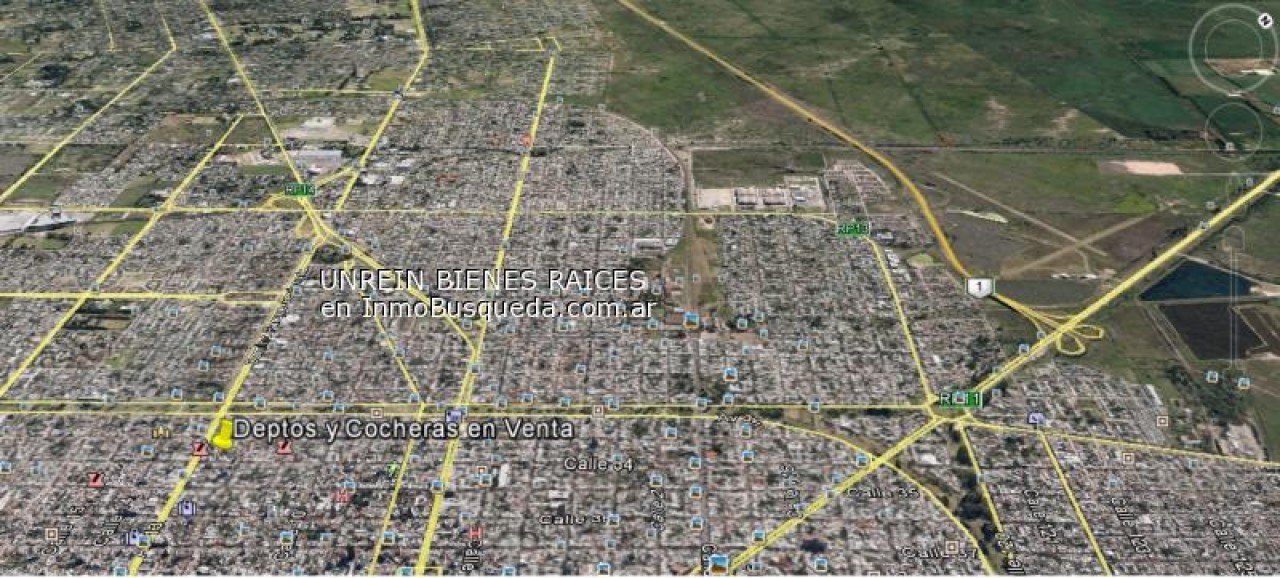The image is an angled satellite view of a suburban or urban area depicting a mix of buildings and natural spaces. The left two-thirds of the image are dominated by densely packed buildings and yellow road networks, indicating a well-developed city or town. In contrast, the upper right section features open green, grassy fields, while the middle right includes a combination of greenery, asphalt areas, and possible road infrastructure, including a labeled Highway 1. Across the middle of the image, there is some overlay text in white that reads, "Unrein Bienes Raíces" and "Inmobusqueda.com.ar." Additional text at the bottom left corner reads "Deptos, Cocheras, and Venta." The language appears to be Spanish, likely indicating the image is from a Spanish-speaking region.